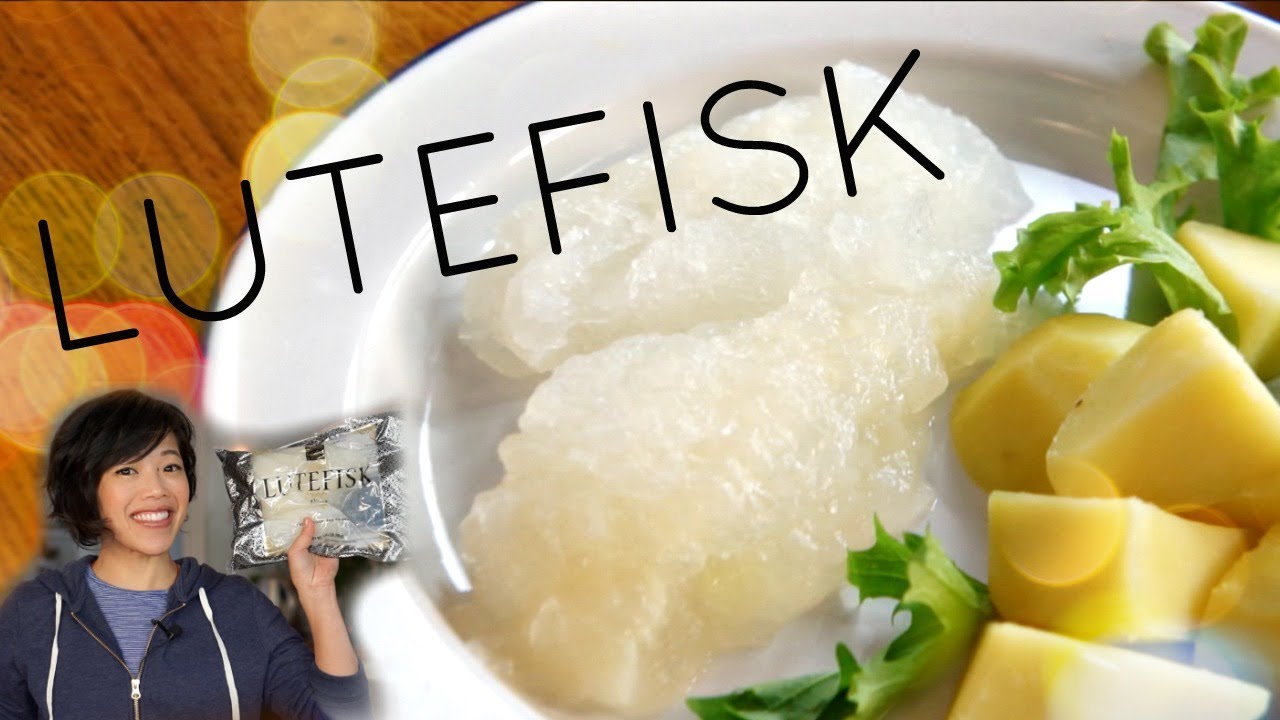In this YouTube thumbnail, an Asian woman identified as the YouTuber EmiMadeInJapan is positioned in the lower left corner. She has a short bob haircut and is smiling warmly. Emi is dressed in a light blue shirt underneath a dark blue zip-up hoodie. She holds a silver package labeled "Lutefisk" in black text.

Central to the image, there is a large white dinner plate placed on a brown wooden table. On the plate is a white gelatinous fish, known as lutefisk. To the right of the fish are yellow cubes, potentially potatoes, and a green leafy vegetable resembling lettuce or parsley.

The title "LUTEFISK" is prominently displayed in black uppercase letters, angling slightly upwards from left to right across the upper portion of the image. Bright yellow light bursts enhance the visual appeal, creating a cheerful and inviting atmosphere.